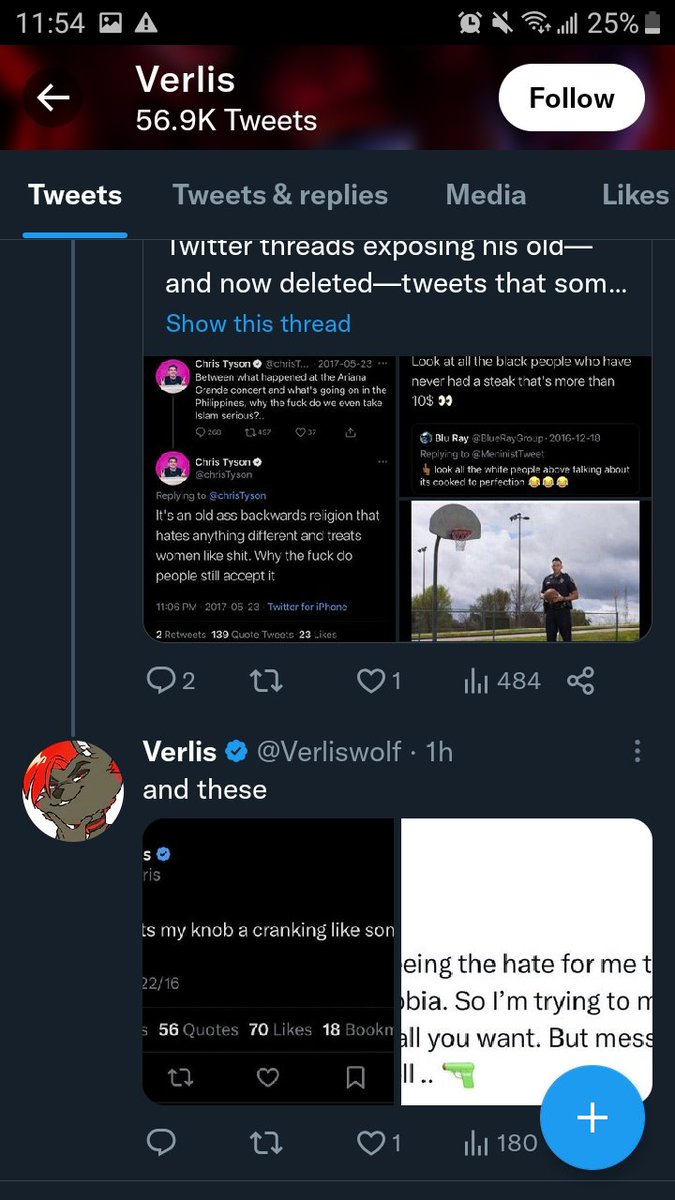The image features a digital interface on a black background. At the top, the display shows "11:54 AM" and a "25% battery" icon. To the left, there is an arrow icon, and next to it, the text "Verlis 56.9k Tweets" is displayed alongside a white "Follow" button. 

Below, the words "Tweets," "Tweets & replies," "Media," and "Likes" appear, with "Tweets" underlined in blue, indicating the current tab. There is text referencing "Twitter threads exposing NIS's old and now deleted tweets…" which is cut off. A button labeled "Show this thread" is visible. 

A small circle with a pink background and a person icon appears along with smaller text next to it. Another image shows the same person with small text again; these elements are inside a black box. To the right, another black box contains three smiley face icons, a small image of a person playing basketball, and various interaction icons including "2 replies," a "heart with 1," "482 lines," and a sideways "V."

Below these, a small circle with a brown character with orange hair and the name "Verlis" appears. It features a blue verified checkmark icon next to "@VerlisWolf," mentioning that the tweet was posted "1 hour ago," followed by an ellipsis icon indicating more options.

Further down, a black and white box with a tiny blue circle and the partially visible phrase “my knob, a cranking like sun,” shows metrics including "56 quotes," "70 likes," and "18 boom." Adjacent to it, some text reading “…being a hate for me so I’m trying to…” and other partially shown phrases.

To the bottom, interaction icons including a "quote mark," "up and down arrow," a "heart with 1," and "180 views" are shown. Finally, there is a large blue circle with a plus mark inside it.